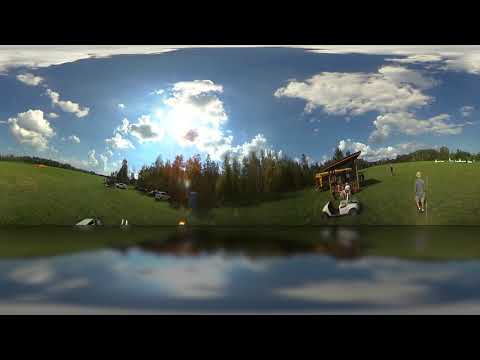A daytime photograph captures a serene golf course scene, where vibrant green grass rolls gently into the distance. Central to the image, a golfer dressed in gray or light blue stands near a white golf cart and a small structure, both located towards the right side of the frame. The golfer faces away from a shimmering lake that occupies the foreground, its surface reflecting a partially clouded, bright blue sky. Scattered across the course are more golfers, enjoying the sunny day amidst clusters of trees that dot the landscape. The image encapsulates the tranquil beauty and the leisurely atmosphere of the golf course, with vividly detailed elements like the sunlit sky, lush greenery, and pristine water enhancing the overall scene.